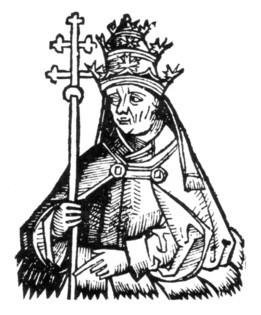The image is a black and white drawing on a solid white background without any borders or text. It depicts an elderly man, who may represent a religious figure or perhaps a pope or king, shown from the waist up. The man is draped in a shawl or cloak fastened near the neck with a strap, and intricate fringe hangs from its bottom. His right hand is holding a staff with a rounded top, adorned with multiple crosses—two crosses extending horizontally, two longer ones extending sideward, and a small cross at the very top. His left hand is bent at the elbow, with the forefinger resting against the front of the staff. He wears an elaborate, multi-tiered crown decorated with intricate points reminiscent of maple leaves and a ball at its apex. The crown and his wrinkled face, accentuated by defining lines, suggest his advanced age.